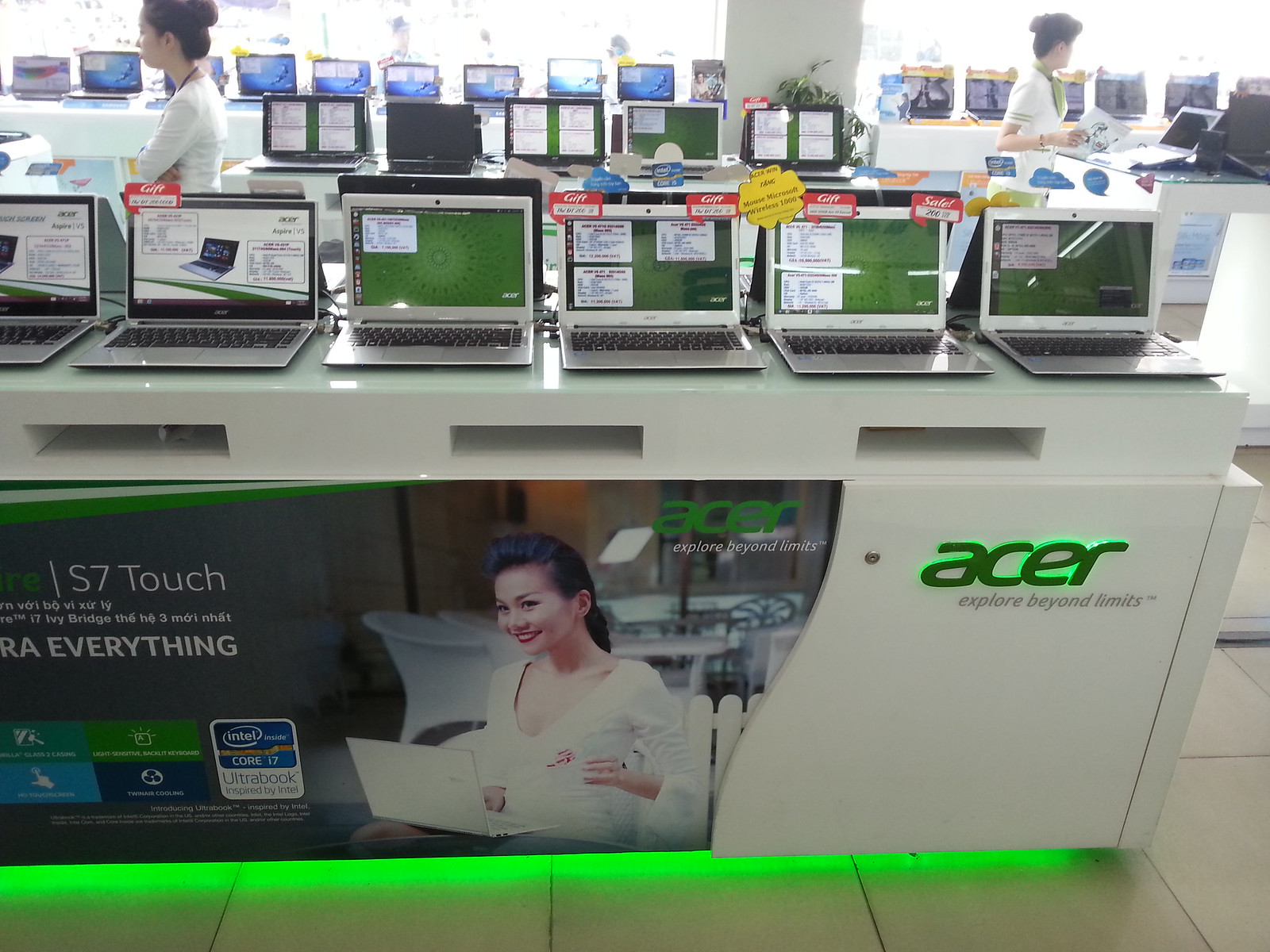This image captures a bustling electronics retail store, specifically focusing on a vibrant display of Acer laptops. The display table, which is white and illuminated by green LED lights from below, prominently features the Acer logo in green neon backlit letters. The brand tagline "Explore Beyond Limits" is also highlighted in glowing green on the display. 

Centered on the table are six open laptops: five fully visible and one partially cut off. These laptops, primarily silver with black keyboards, have screens displaying a mix of white and green backgrounds along with various informative stickers, showcasing their features and specifications. Most of the stickers include details like "S7 Touch" and the Intel Core i7 logo alongside other colorful stickers in green, blue, and white.

An advertisement positioned to the left of the table presents an Asian woman in a white blouse holding an Acer laptop on her lap. This ad features additional text, such as "S7 Touch" and the Intel Core Ultrabook logo, although some of the informative text is cut off at the picture's edge.

In the background, the store's activity continues with numerous other laptops displayed on tables and customers browsing, accompanied by two store employees dressed in white shirts. The blend of the bright green Acer branding, strategic lighting, and the dynamic retail environment highlights the emphasis on Acer products in this lively store setting.